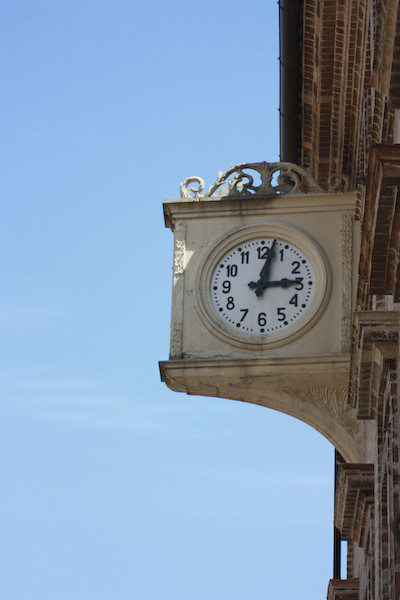This photograph, taken in daylight, showcases a large, sculpted clock affixed to the side of a brick building with brownish bricks. The clock, framed in a beige or cream-white frame, features intricate scroll work on its top and a half arch at the bottom. It extends one to two stories high from the building. The clock's circular face has a white background with black Arabic numerals marking every hour and smaller dots indicating the minutes in between. The time displayed is 3:02, with the little hand pointing near 3 and the big hand just past the 12. The blue sky dominates the left side of the image, enhancing the prominence of the clock against the brick building.